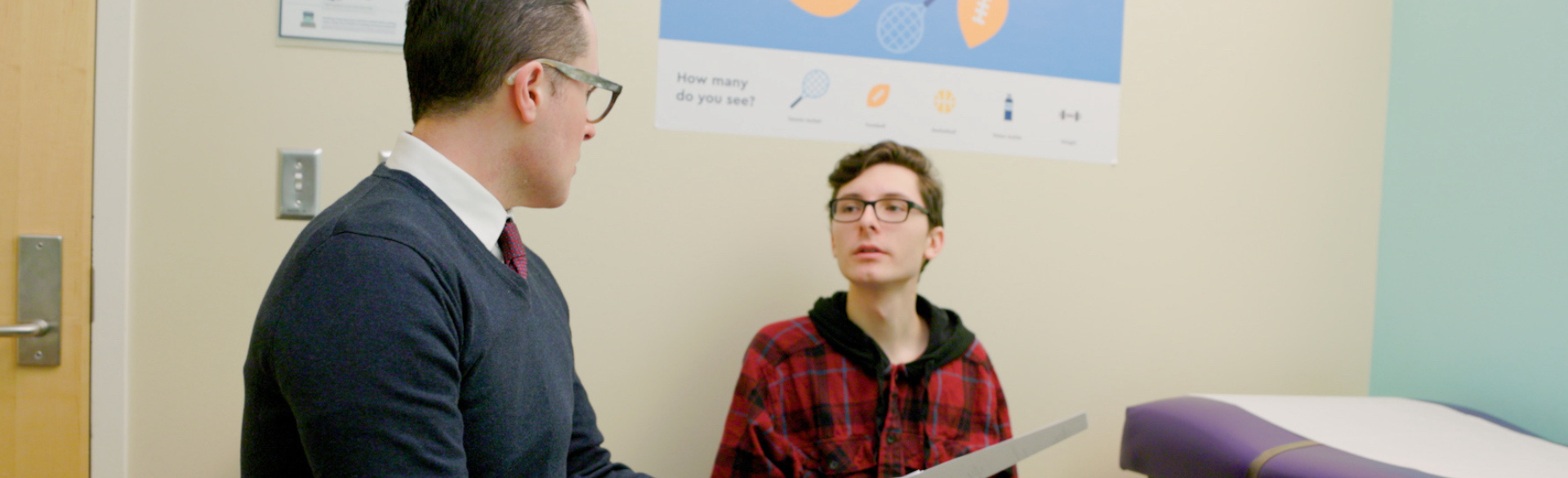In this landscape-oriented photograph, an interaction between two males is captured inside a room that resembles a doctor's office. The image's width is significantly longer than its height. On the left, there is a partial view of a light brown wooden door with a metallic handle. The adjacent wall is cream-colored and features several partially visible posters. To the right, a segment of another wall, painted in a light blue or seafoam green, can be seen.

Central to the image are two Caucasian males, both wearing glasses and engaged in conversation. The man on the left has black hair, wears a white shirt under a dark gray or navy sweater, and a purple tie. He appears to be speaking and looking towards the second person. This second individual, positioned slightly behind and to the right of the first, is a younger male, possibly a teenager, with brown hair, wearing a black and red jacket. He seems to be listening attentively to the older man.

In the background, the room's setting further hints at a medical environment – a purple examination table with white paper is partly visible, alongside bits of a blue, orange, and white poster. The scene depicts a focused moment of communication, possibly involving instructions or discussion, within a clinical or educational context.